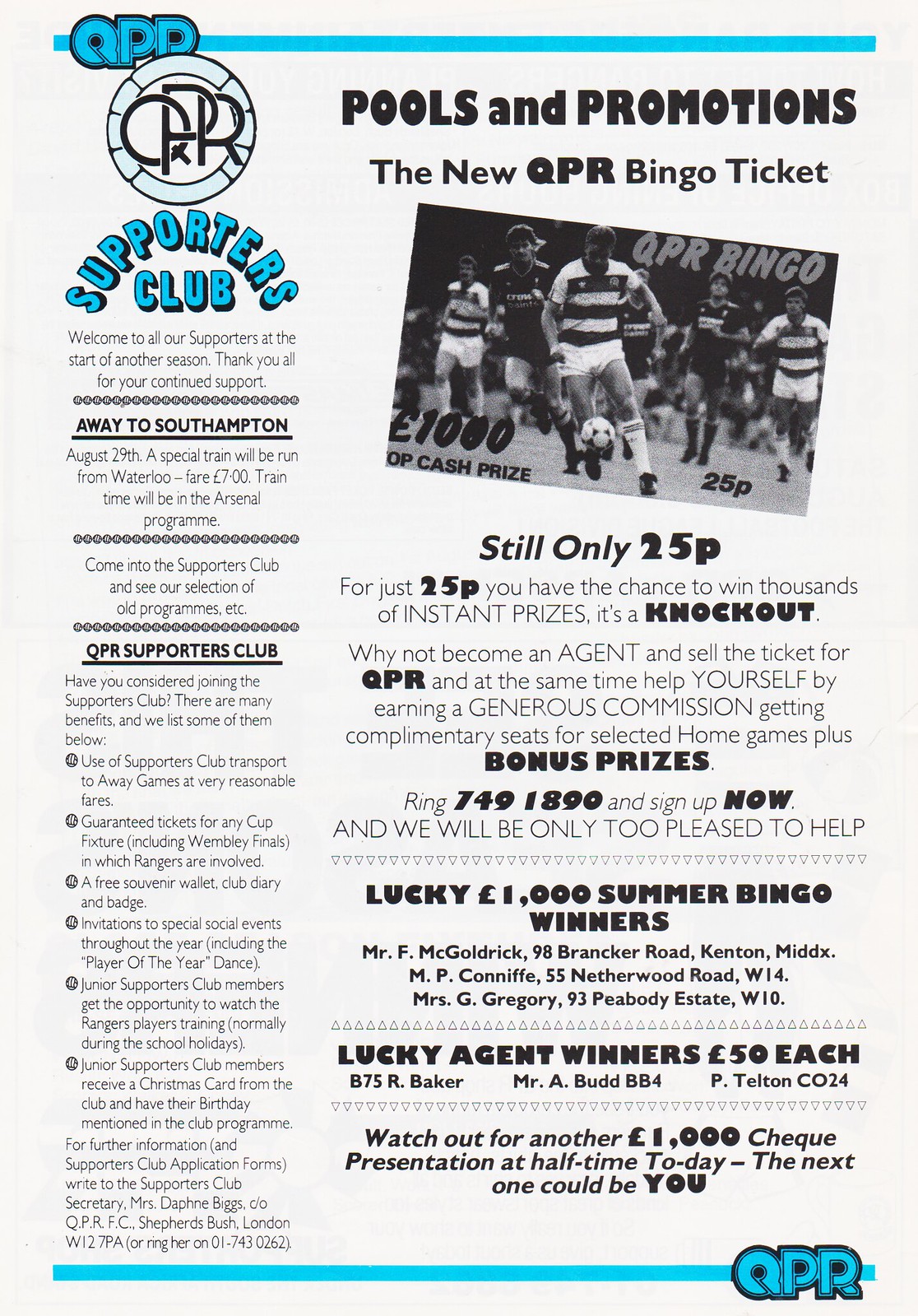This flyer is an old British football advertisement for the QPR (Queen's Park Rangers) Supporters Club. It features a predominantly black and white design with light blue accents including a top and bottom border and bold blue capital letters “QPR” in the upper left corner. Beneath this, in black, is a larger version of “QPR” followed by “Supporters Club.”

The left-hand column welcomes supporters to the new season and thanks them for their continued support, mentioning an away game to Southampton and a special train from Waterloo available for 7 pounds. The flyer details benefits of joining the Supporters Club such as discounted transportation to away games, guaranteed tickets for fixtures including finals, free souvenirs, and invitations to special events. Junior members can watch Rangers' training sessions and receive Christmas cards and birthday mentions in the club program.

On the right side, the flyer promotes the new QPR bingo ticket, highlighting a photo of men playing soccer. For only 25p, participants have a chance to win thousands of instant prizes. The flyer includes a call to become an agent to sell tickets, offering generous commissions, complimentary seats for selected home games, and bonus prizes. It also lists previous prize winners and mentions an upcoming £1000 check presentation at halftime.